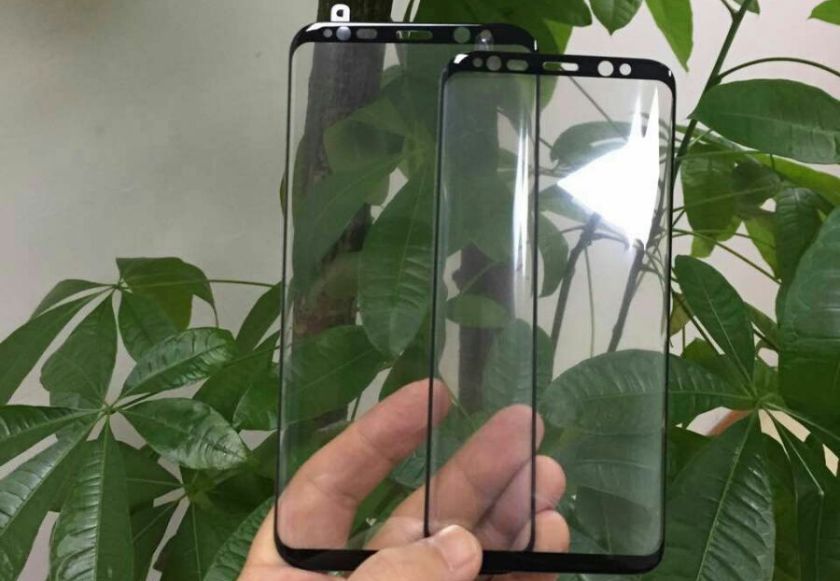A man's left hand holds up two clear phone screen protectors of different sizes in this photograph. These protectors feature black borders at the top, bottom, and sides, with cutouts for cameras, microphones, and other sensors, and are otherwise transparent with a slight haze. The hand appears to be of fair complexion, with visible fingers and thumb. The protectors are held against the backdrop of a large indoor Chinese money tree, characterized by its two sizable trunks and numerous glossy, long, narrow green leaves. The background consists mostly of the foliage, except for the top left corner, where a gray to white blank wall is visible. The image has a low quality and notable glare on one of the protectors, suggesting the lighting comes from the back right.